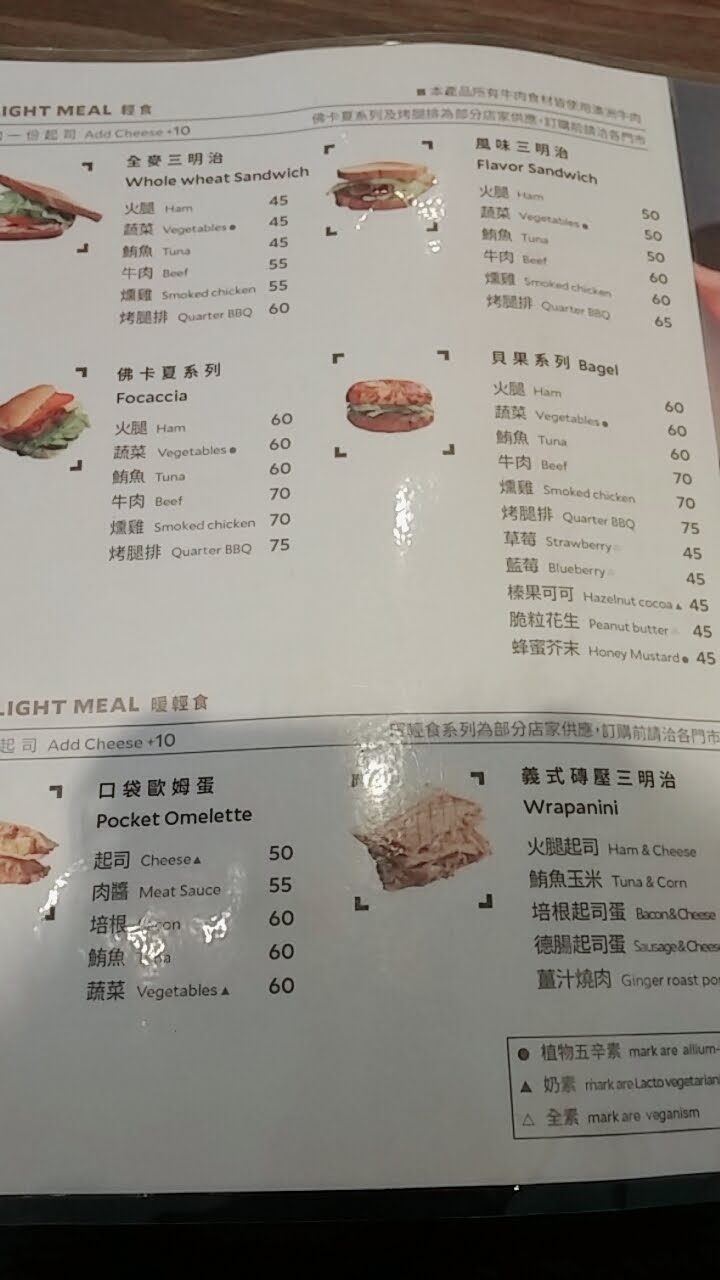The image displays a glossy, laminated page from a restaurant menu dedicated to sandwiches. The layout features six images, each depicting a different type of sandwich, accompanied by their names. In the top left corner, there is an image of a Whole Wheat Sandwich. Directly below it, the second sandwich on the left is a Focaccia Sandwich. The sandwich in the bottom left corner is labeled as a Pocket Omelette.

On the right side, starting from the top, we see an image of a Flavor Sandwich. Directly below that, there is a Bagel Sandwich, represented with a clear picture. The final sandwich featured on this page, situated in the bottom right corner, is a Rapanini Sandwich. The arrangement and detailed visuals provide a comprehensive overview of the sandwich offerings available at the restaurant.